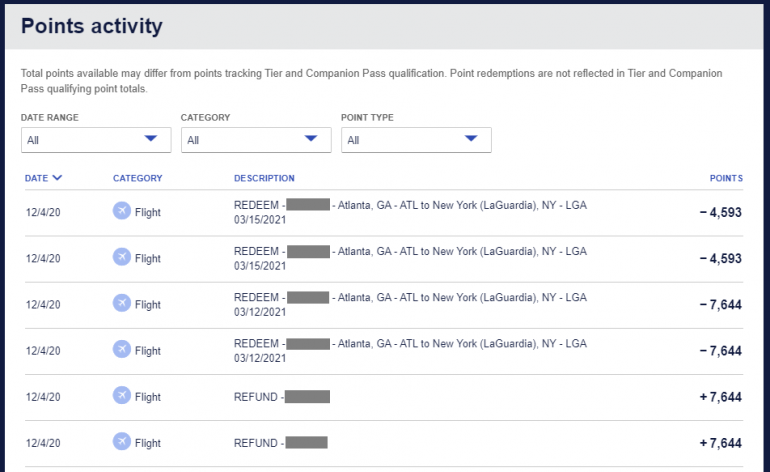The image is a detailed screenshot displaying the activity points for someone's rewards membership, likely related to a credit card or frequent flyer program. The image has a horizontal, landscape orientation with thick black borders on the left, right, and top edges.

At the very top, there's a gray bar with the title "Points of Activity" in black text, followed by a white section with an important note: "Total points available may differ from points tracking tier and companion pass qualification. Point redemptions are not reflected in tier and companion pass qualifying point totals."

Below this, there are search options set in white drop-down menus, currently displaying settings for "Date Range," "Category," and "Point Type," all defaulted to "All."

Following the search options, a list of point activity entries is shown, all dated 12/4/20 within the flight category. The descriptions provide detailed information about each activity:

1. **Redeem Atlanta, GA (ATL) to New York, LaGuardia, NY (LGA) - 3/15/2021** 
   - **Points**: -4,593

2. **Redeem Atlanta, GA (ATL) to New York, LaGuardia, NY (LGA) - 3/15/2021** 
   - **Points**: -4,593

3. **Redeem Atlanta, GA (ATL) to New York, LaGuardia, NY (LGA) - 3/12/2021**
   - **Points**: -7,644